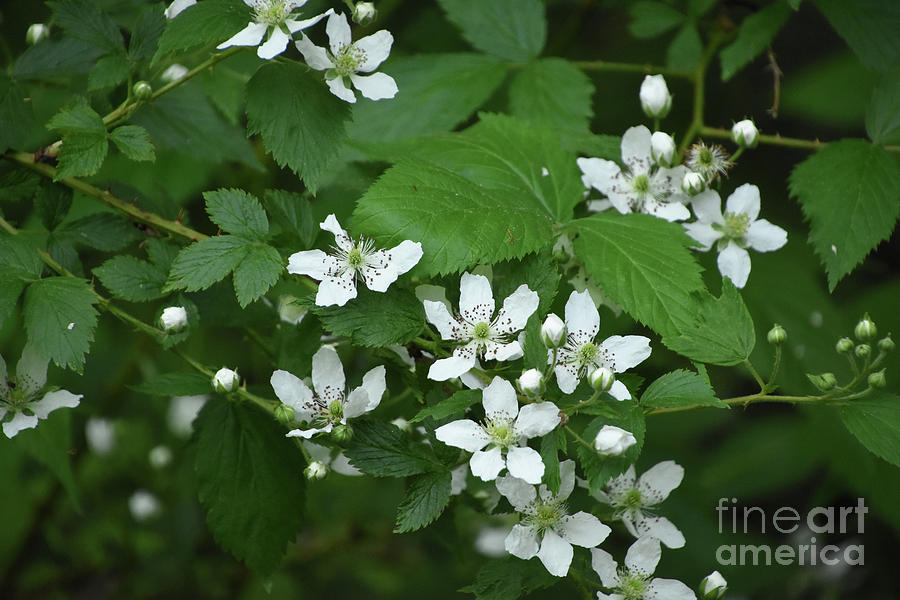The image captures a close-up view of a thorny blackberry vine adorned with vibrant green leaves and delicate white flowers. Most flowers have five petals and prominently feature brown, pollen-laden stamens extending up to half an inch from their centers. Some flowers appear fully bloomed, while a few remain unopened, resembling tiny cotton bulbs. Thorns and green vines can be seen in both the upper left and upper right corners of the image. The green background is artfully blurred to emphasize the plant's intricate details, and in the bottom right corner, a watermark reads "Fine Art America."